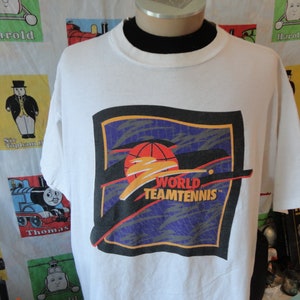The image captures a detailed close-up of a headless mannequin dressed in a white graphic t-shirt, layered over a black long-sleeve undershirt. The t-shirt features a central box logo that reads "World Team Tennis," with "World" in orange and "Team Tennis" in yellow, accompanied by a yellow zigzag design. A blue, globe-like grid pattern can be seen in the background of the logo. The frame around the logo is black, against a blue wash background. The mannequin is presented against a backdrop that includes numerous flyers and a wall tapestry adorned with characters from "Thomas the Train," including the conductor and other trains from the show. The scene is bathed in natural light from the left side, and the mannequin’s right sleeve is visible while the left one appears to be tucked back.